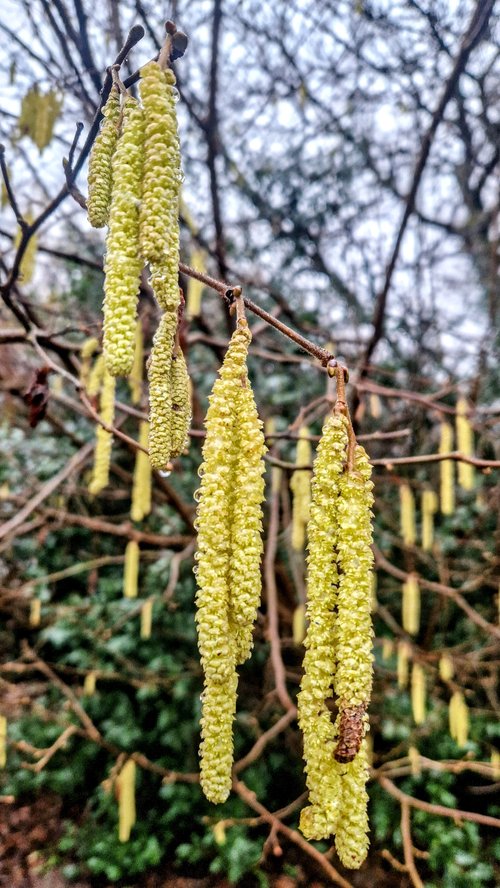This detailed color photograph captures a close-up of tree limbs adorned with long, drooping clusters of pale yellow seed pods or flowers. The camera focuses primarily on three prominent clusters, resembling cylindrical rods or fluffy, yellow worms, hanging gracefully. Each cluster appears interconnected at the top, with a few showing brown tips, adding to the visual interest. These clusters, evocative of corn cobs, descend from the branches with a pale yellow to greenish hue, creating a striking contrast against the bright, white sky in the background. Out of focus, additional clusters and bare limbs stretch across the top of the image, suggesting a seasonal setting of either spring or fall. The lower part of the image reveals some green, possibly from other vegetation or ground cover.